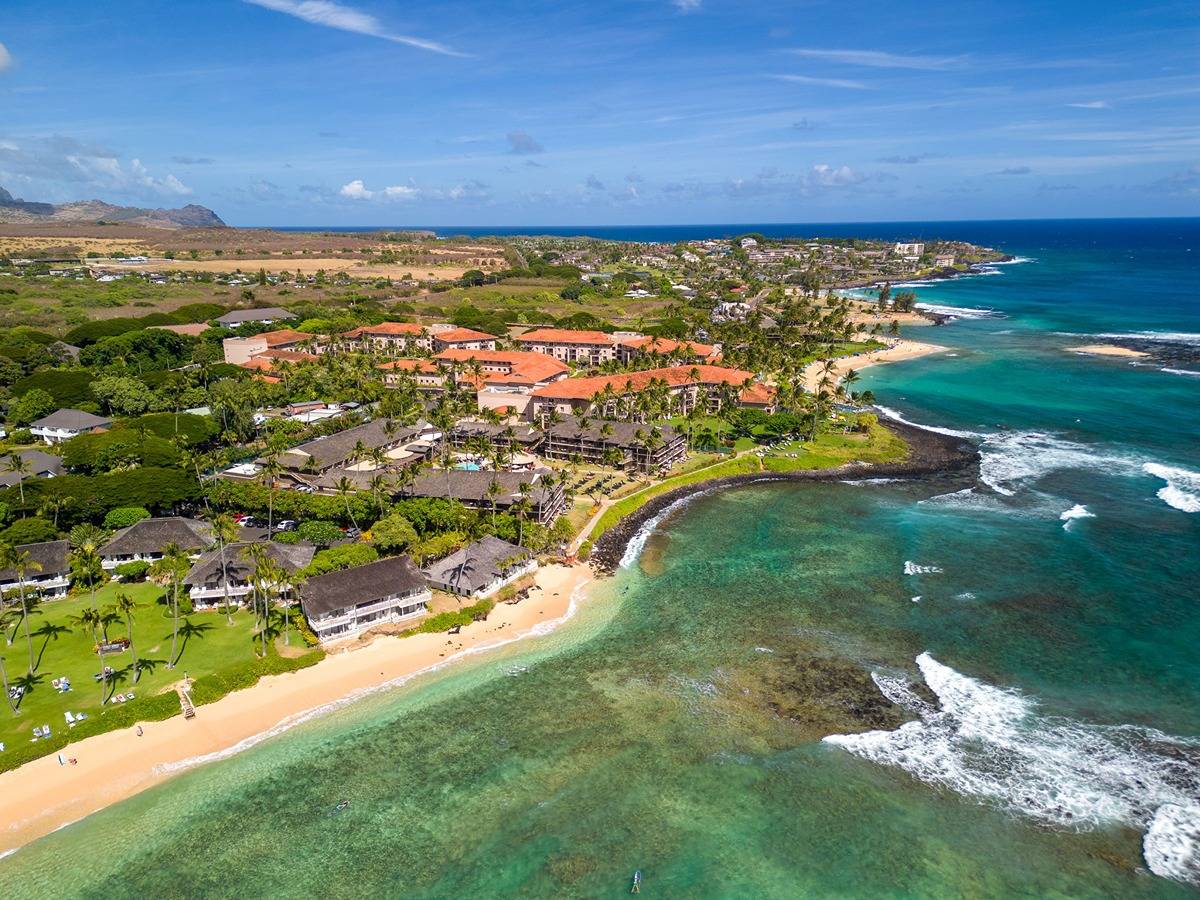This aerial, or drone-captured, photograph beautifully depicts a coastal area likely situated on a tropical island. The scene showcases an expansive beach beside deep blue and green hues of ocean waters under a clear, sunny sky. Scattered high clouds add to the picturesque backdrop.

Dominating the shoreline is a developed area reminiscent of a resort, with several pools and seating areas indicating luxurious accommodations. The resort features a mix of architectural styles: on the left, buildings with dark gray thatched roofs, and on the right, more modern structures with cream-colored walls and reddish-orange roofs. An abundance of palm trees punctuates the lush greenery surrounding the resort, further emphasizing the tropical setting. This vibrant, idyllic locale suggests a perfect vacation spot, possibly in Hawaii or a similar tropical destination.